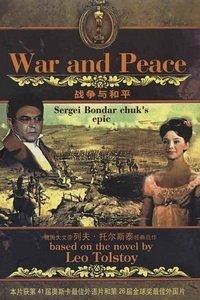The image depicts a cover, possibly of a book or a movie poster, featuring a composition of both dark and light colors. The central text prominently displays "War and Peace" in bold orange letters. Below that, in dark black text, it states "Sergei Bondarchuk's epic." The cover is split with the left side showing a man and the right side portraying a woman dressed in pink with her hair up. The background includes a blurred image, potentially a battlefield scene. There is also a bronze crest symbol at the top. Additionally, the cover contains Chinese characters beneath the "War and Peace" title and at the bottom. The text at the base reads "Based on the novel by Leo Tolstoy."